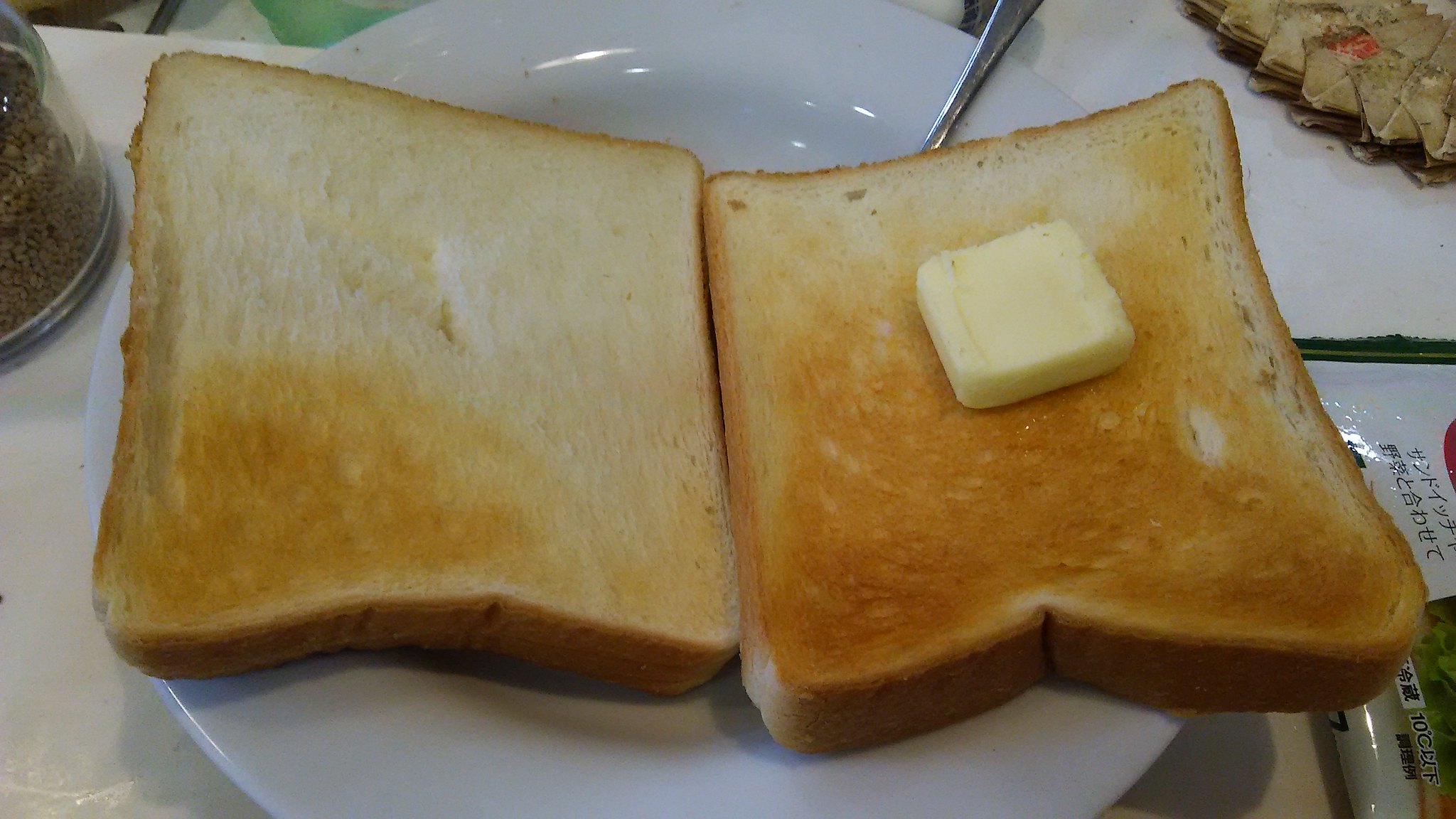This image captures a close-up of two slices of lightly toasted white bread, positioned side-by-side on a round white plate. A cold, unmelted square of butter rests prominently on the right piece of toast. The plate sits on a white table, and a small fork is partially visible at the top right corner, mostly obscured under the toast. In the background, on the left side, there is a glass container filled with black granules, likely coffee. To the right edge of the image, there is a piece of paper with writing in an East Asian script, possibly Chinese or Japanese. The overall composition is simple and minimalist, focusing on the everyday breakfast scene.